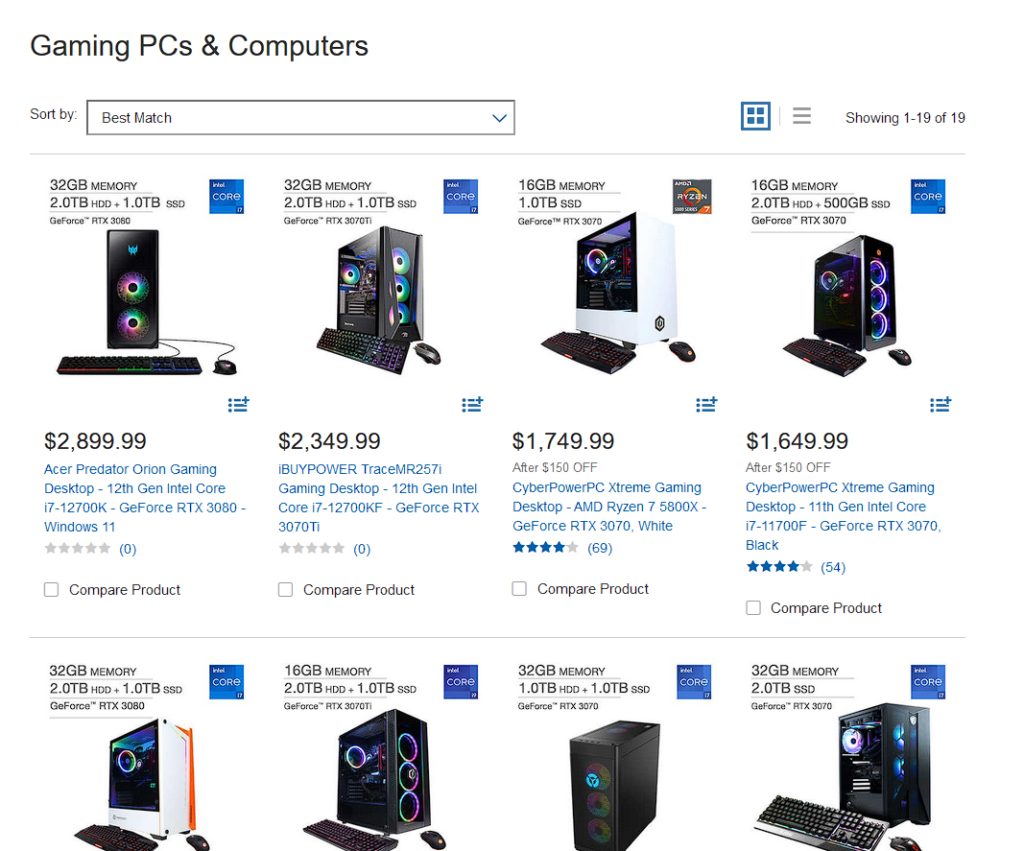This image showcases a retail webpage dedicated to gaming PCs and computers. At the top of the page, on a white background, the words "Gaming PCs and Computers" are prominently displayed in black text. Adjacent to this heading, there's a "Sort by" section with a dropdown menu currently set to "Best Match."

The main body of the page features images and details of eight different computer towers, all designed for gaming. Each tower's image is topped with crucial hardware specifications, including system memory and processor information, alongside their respective processor logos. Below each image, the pricing details are provided clearly.

The first computer listed is the "Acer Predator Gaming Desktop," followed by the "iBuyPower TraceMR25i Gaming Desktop." Next is the "CyberPowerPC Extreme Gaming Desktop," and another model simply described as the "CyberPower Extreme Gaming Desktop." Unfortunately, the descriptions for the remaining four towers are cut off and not fully visible in the image.